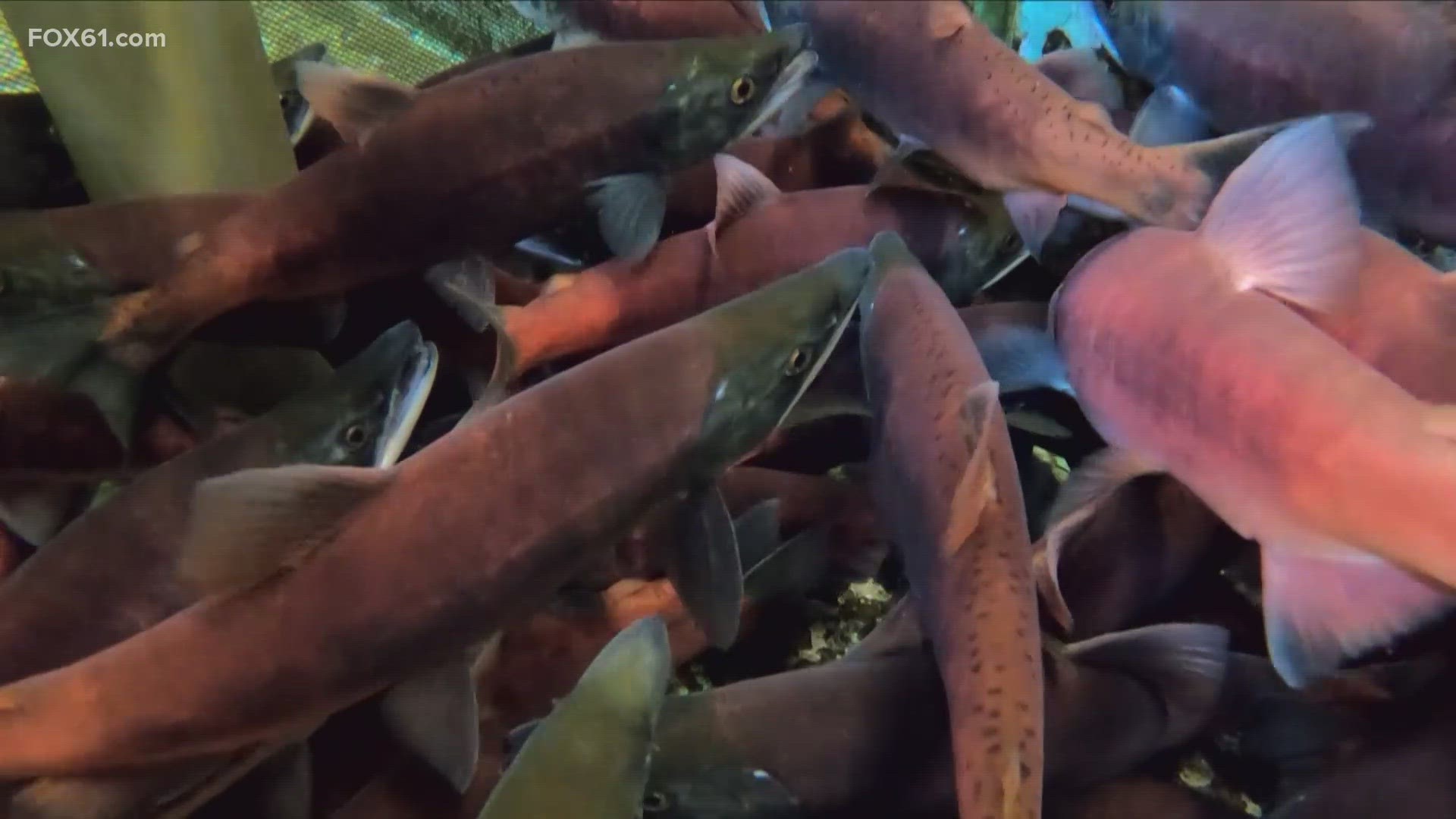In this underwater scene, a group of fish, likely pink salmon or a similar trout species, swim in crystal-clear water. The fish are characterized by their pinkish-red bodies, which transition to a rust color, with dark green heads and fins. Their eyes have a black pupil surrounded by a yellow ring, and some mouths are slightly open. The water is exceptionally clear, suggesting it might be a clear brook, stream, or possibly a lake. Clustered together in a dense school, the fish dominate the frame, with 10 to 12 easily visible and potentially more at lower levels. The image also contains the text "Fox61.com" in the upper right, possibly indicating a nature segment from the TV channel. The environment is vibrant and reveals intricate details of the fish, including speckles and scales, set against the clarity of the water.